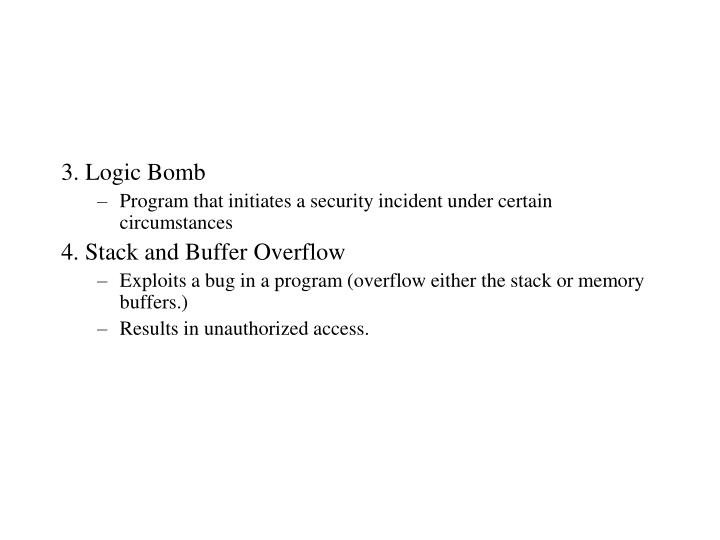The image features black text on a white background, prominently positioned in the center with ample white space above and below. It appears to be part of an educational slide, likely derived from an academic or training presentation. The content includes:

1. "3. Logic Bomb." - This title is in black text, with capitalized initial letters for "Logic" and "Bomb". Beneath it, an indented bullet point states: 
   - "Program that initiates a security incident under certain circumstances."
   
2. "4. Stack and Buffer Overflow." - Similar to the former, this title is numbered "4" followed by a period, with each main word capitalized except "and". The detailed points under this title include:
   - "Exploits a bug in a program (overflow either the stack or memory buffers)."
   - "Results in unauthorized access."

The text is well-spaced, clear, and neatly centered, enhancing readability on the stark white background. This minimalistic design emphasizes the educational content, making it easy to follow and visually appealing.